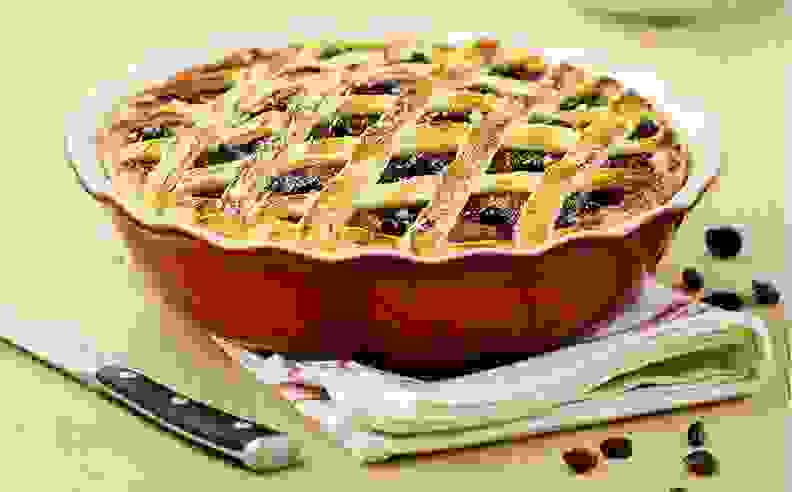The image depicts a heavily pixelated blueberry pie with a lattice crust, visible through which the blueberry filling slightly oozes out. The pie is situated in a red pie pan with a white interior, resting on a folded white kitchen towel adorned with green ends. A knife with a dark handle featuring three silver dots lies to the left of the pie, its blade angled slightly to the left. Scattered around the pie are eight blueberries, four in front and four to the right. The background primarily consists of a mix of light and dark green, rendered in blocky, pixelated squares. This gives the impression of a digitally altered, almost painted effect.